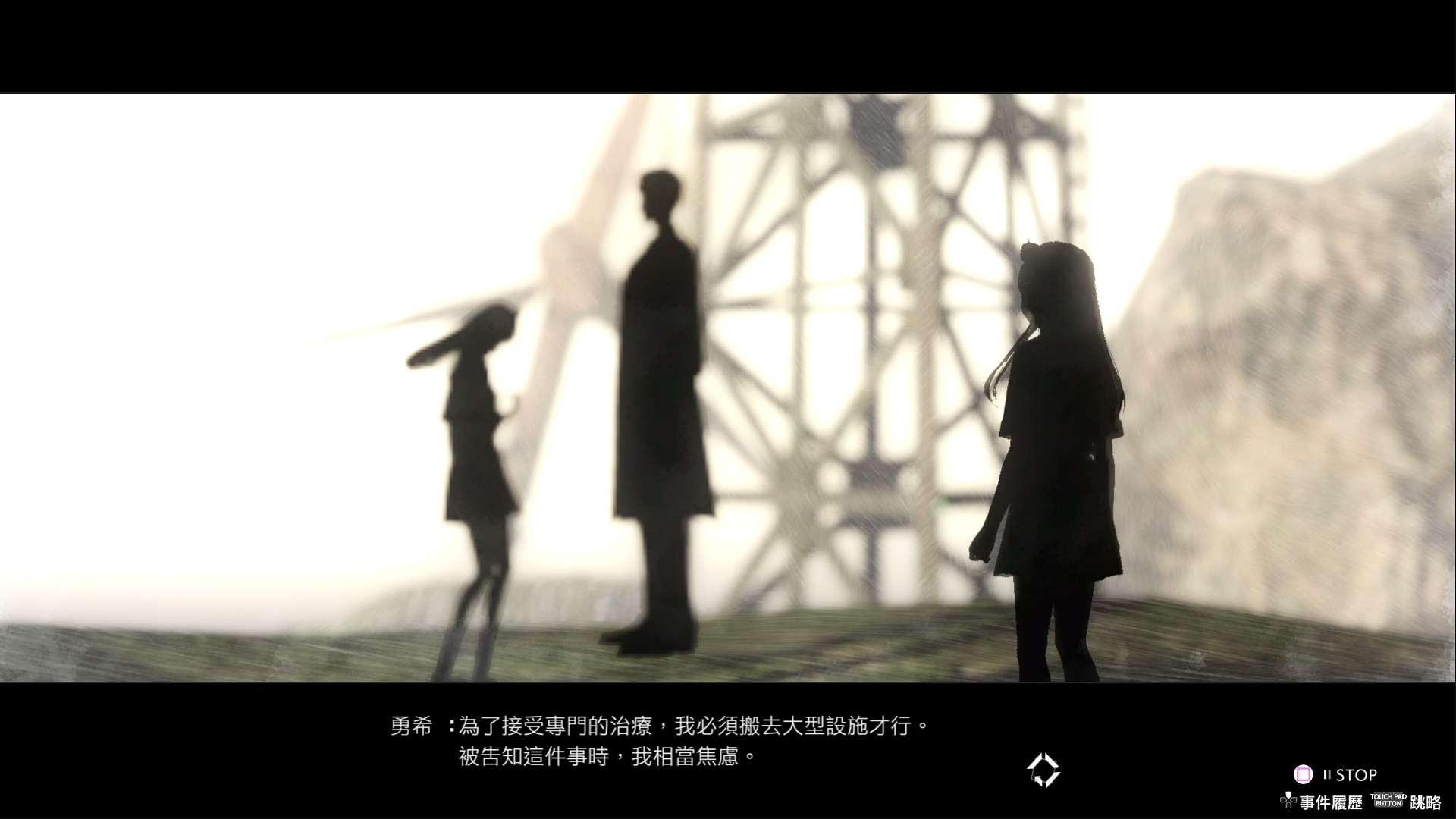The image is a digital screenshot from a video game, featuring Japanese subtitles at the bottom. At the bottom right, the English word "STOP" is visible, along with references to a "touchpad button" near a diamond-shaped control area, which is partially blacked out. The scene is set outdoors on a cliffside, showcasing a man and a woman standing near a large radio tower or windmill in the background, with rocky mountains to the right. In the foreground, a little girl faces the man. All characters are silhouetted, making it difficult to discern specific details about their clothing. The overall color palette includes shades of black, white, gray, and green, giving the image a somewhat blurred appearance.